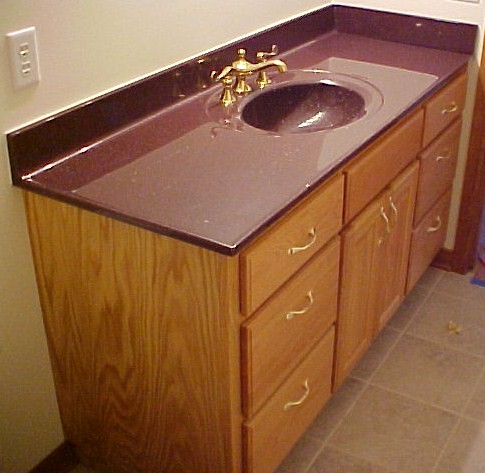This photograph showcases an elegantly designed bathroom vanity, featuring a rich maroon quartz countertop seamlessly integrated with a matching basin sink. The sink is adorned with gold, intricately designed fixtures, including a faucet reminiscent of Aladdin's lamp, adding a touch of opulence. The vanity is set against off-white walls that provide a subtle contrast, highlighting the medium reddish wood of the drawers and cabinet beneath. The floor is tiled in a beige hue, complementing the overall color scheme. On the far left end of the vanity, an electrical outlet is embedded in the wall, which also showcases the room's wooden trim and a visible wooden door frame. The drawers and cabinet handles gleam in gold, matching the faucet and enhancing the luxurious feel. There appears to be a rug near the entrance, though it is partially obscured and not fully discernible in the image.